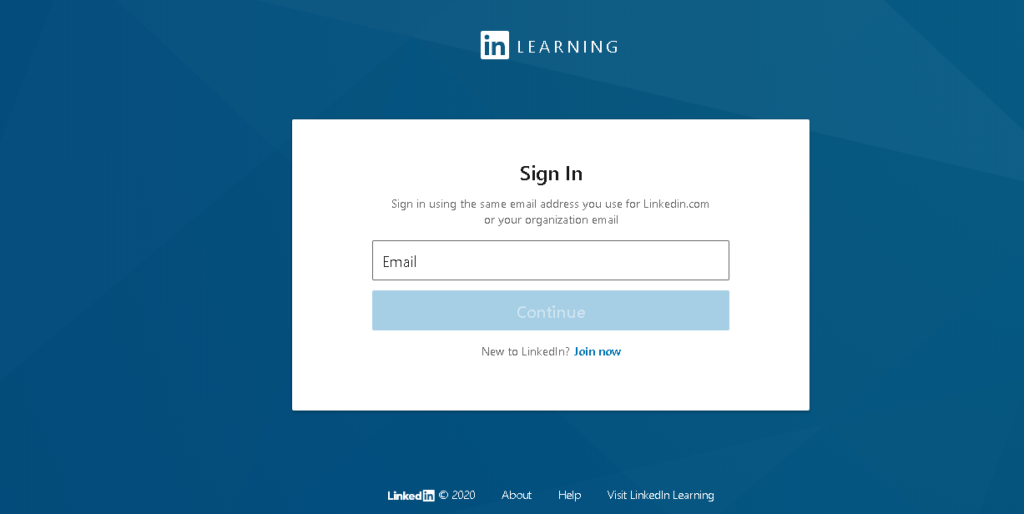The image depicts a predominantly blue background with an overlay pop-up box prominently displaying the text "In Learning." This indicates a LinkedIn program designed for educational purposes. The pop-up prompts users to sign in by entering their email information into the provided field. Below this, there is a blue button labeled "Sign In." Additionally, there is a call-to-action message encouraging new users to join LinkedIn, accompanied by a yellow button that says "Join Now." At the very bottom of the image, there is a footer with white text stating "LinkedIn 2020" along with links for "About," "Help," and "Visit LinkedIn Learning." The overall layout does not specify what the learning content entails, keeping the focus solely on the act of learning. All the text within the image is written in white, except for the interactive elements, which are highlighted in blue and yellow for emphasis.